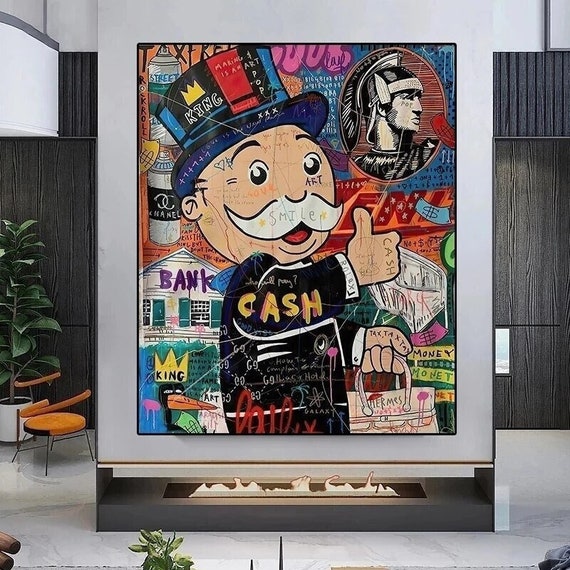This vibrant and detailed piece of modern artwork, displayed prominently in a stylish, modern home with a visible fireplace, recreates the chaotic and dynamic essence of graffiti on a large canvas. The focal point is a pop art depiction of the Monopoly mascot, Mr. Monopoly, adorned with a top hat labeled "King" and featuring a crown. The piece includes numerous references to financial themes, with words like "cash" repeated throughout and "tax, tax, tax" displayed on his raised thumb. Mr. Monopoly gives a thumbs up while holding a Hermes bag, and the artwork is embellished with various eclectic elements including a Roman soldier, a bird wearing a crown, and a small structure labeled "BANK" with purple letters and blue shutters. Additionally, there are nods to famous names with "Monet" spelled out, a Chanel spray bottle, and the phrase "Rock and Roll." The composition is vibrant and busy, reflecting the messy, layered style typical of graffiti art.